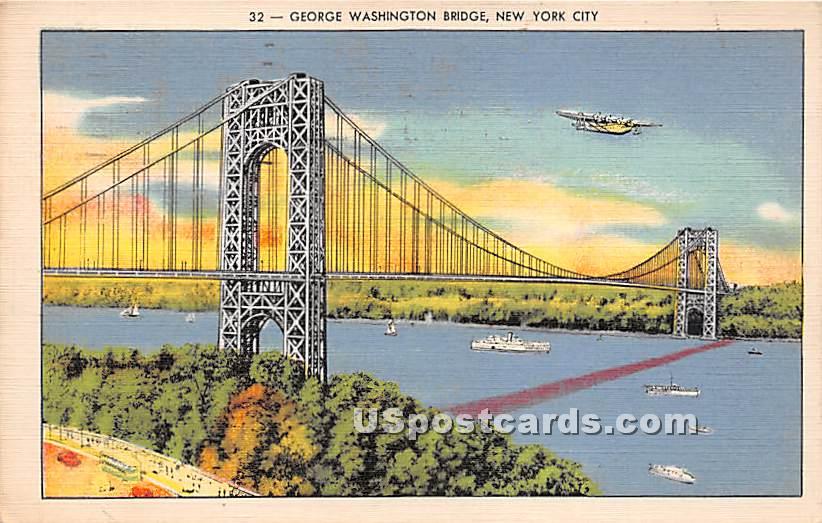This vintage-style, horizontal postcard, bordered by a dark cream (or peach) outline, features an illustration labeled "32-George Washington Bridge, New York City" at the top center in black font. The bottom right corner displays a watermark reading uspostcards.com. The central image depicts the iconic George Washington Bridge, characterized by its massive towers and extensive cables stretching across the Hudson River. The bridge is primarily depicted in white and black, possibly suggesting a steel, silver-toned structure. The scene is set against a vivid, late-day sky transitioning from deep blue at the top to yellow and orange hues toward the left, signifying sunset. A plane soars through the top right corner of the image. Beneath the bridge spans the Hudson River, featuring a red shadow cast across the water. Several white boats dot the river, which is flanked by lush green vegetation. In the foreground on the left, a street with a thick sidewalk and numerous pedestrians is partially obscured by trees. The combination of colors and elements gives the postcard an older feel, reminiscent of the 1970s or 1980s.